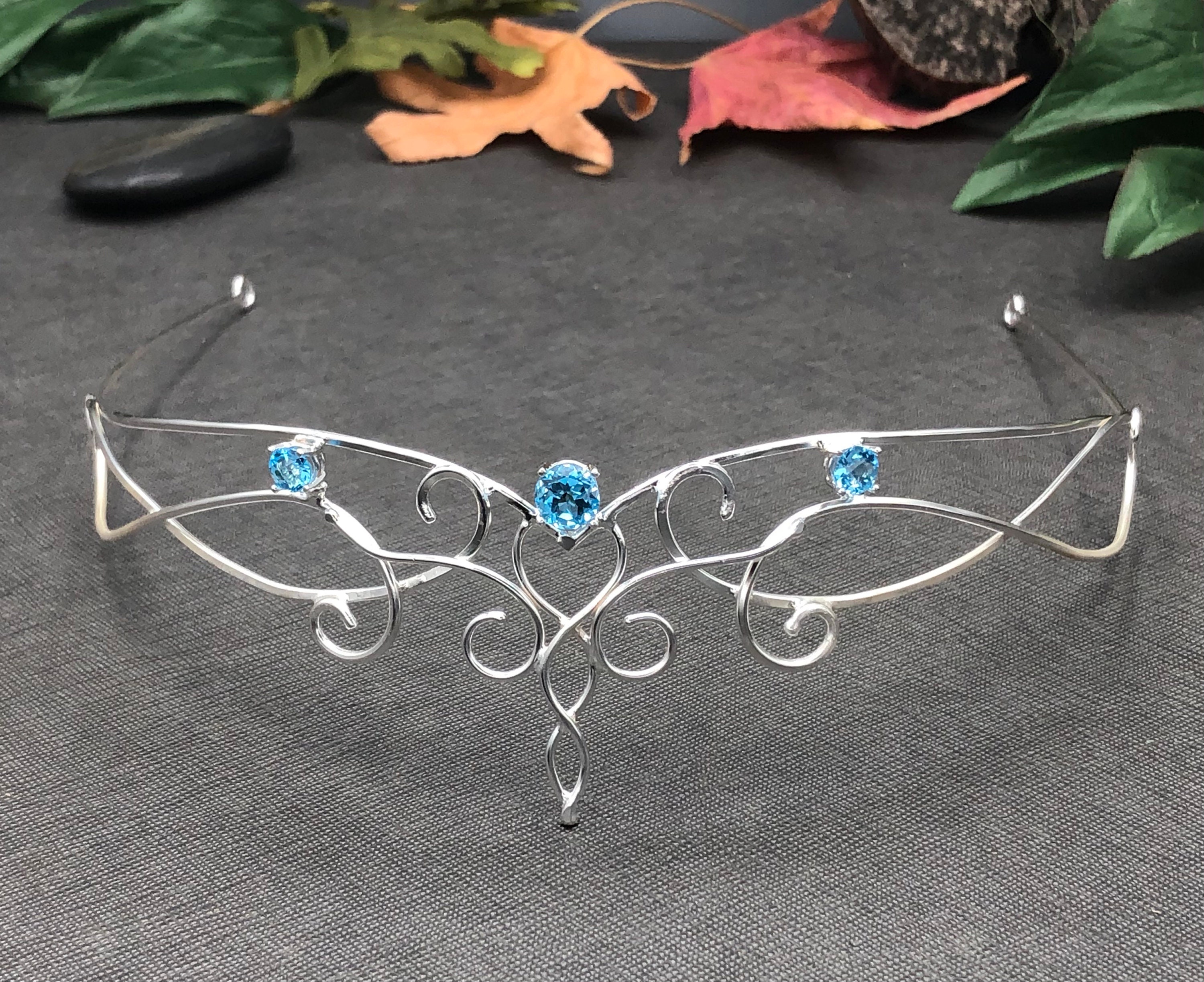This close-up image features an intricate, elegant silver tiara that appears almost like a tight clutch necklace, set against a gray burlap background. The elaborate filigreed silver design is adorned with three light blue stones, one centrally positioned and two on either side. The tiara's delicate construction includes four loops along the bottom and a vertical ornamentation resembling the intertwining snakes of a caduceus, gracefully descending towards what would traditionally be the nose area. Straight posts extend backward to hold the piece in place.

The symmetrical floral pattern of the tiara further enhances its refined craftsmanship. The backdrop of the shot showcases autumnal leaves at the top, in shades of yellow, orange, red, and green, accompanied by a smooth, oval-shaped polished black stone on the top left corner. This juxtaposition of the dainty, sparkling tiara against the rustic, textured gray fabric and vibrant, seasonal elements creates a striking and detailed composition.